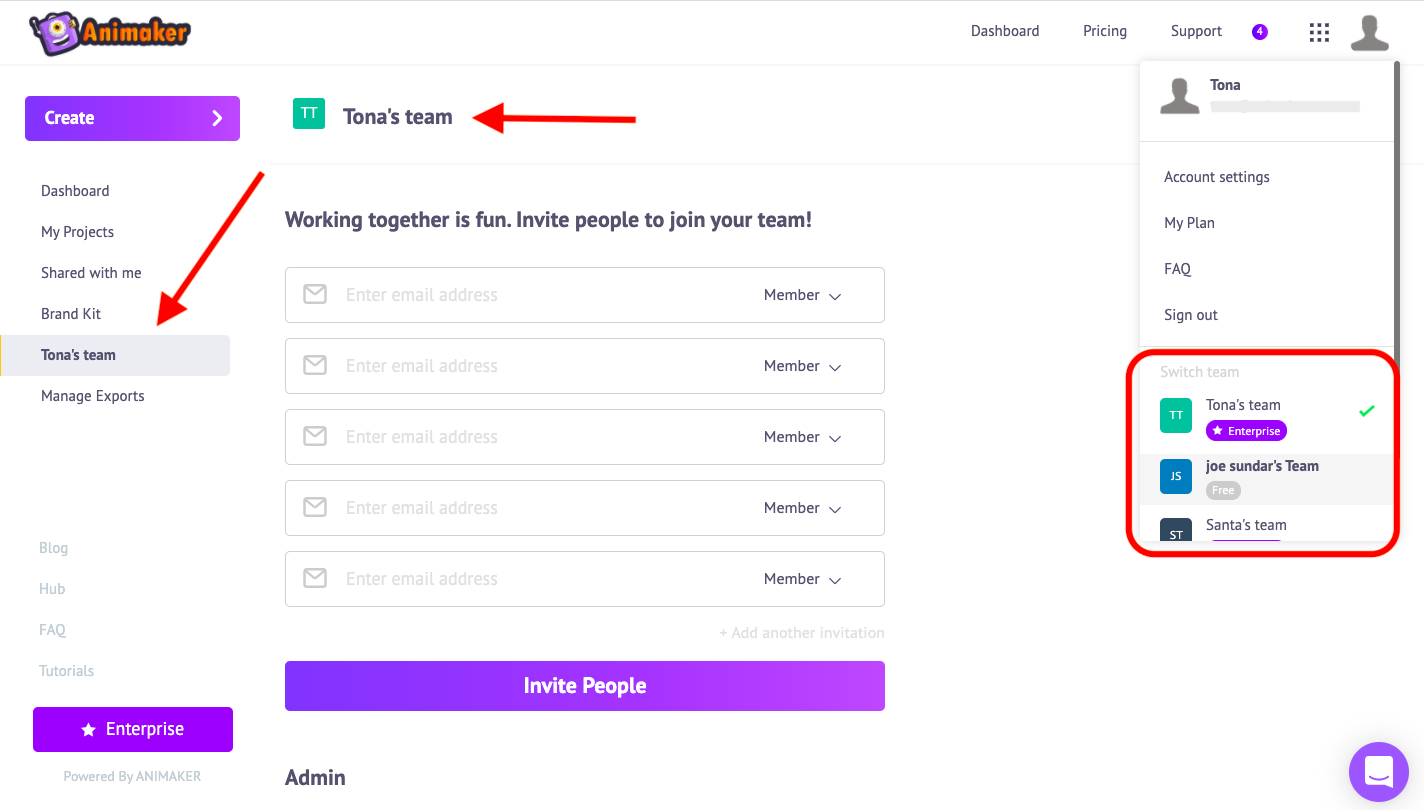The background of the image is white. In the upper left-hand corner, there’s an image of a cute purple monster with one eye. Next to the monster, "Anna Makea" is written in bold orange text with a purple outline. To the right of that, in black text, it says "Dashboard Pricing Support." Nearby, there’s a purple circle with a white number "4" inside it.

On the left side of the image, there’s a purple rectangle with the word "Create" written in white. Below this, in black text, it lists "Dashboard, My Project, Shared With Me, Brand Kit, Toner's Team," all enclosed within a gray box. A red arrow points to this list. Beneath that, also in light gray, it says "Manage Exports." Following this are the words "Blog Hub, FAQ, Tutorials."

Further down, there is another purple rectangle containing a white star, and it says "Enterprise" in white text. Below this, it states "Powered by Anna Makea."

Towards the middle of the image, there’s a green square with white "TT" written inside. Next to the square, in black text, it says "Toner's Team," with a red arrow pointing to it. A thin gray line spans across the image. Below this line, in black text, it reads "Working Together is Fun. Invite people to join your team." Followed by five input fields labeled "Enter Email Address," and these fields have an accompanying "Member" tag.

At the bottom of these fields, there is a purple rectangle with the phrase "Invite People" written in white. Underneath this, in black text, it says "Admin."

On the right-hand side of the image are various options labeled in black text: "Toner Account Settings, My Plan, Frequently Asked Questions, Sign Out." There’s a red rectangular box surrounding "Toner's Team, Joel Sundar's Team, and Santa's Team.”